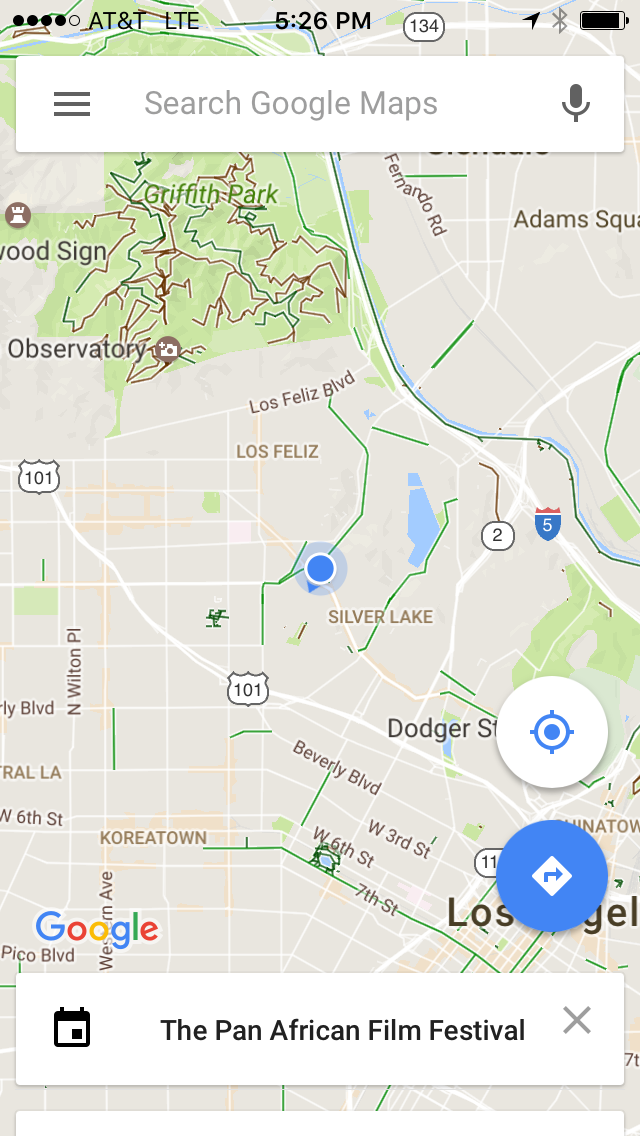This image depicts a smartphone screen displaying Google Maps. In the top left-hand corner, there are five circles, four of which are black, indicating signal strength, followed by the labels "ACMC" and "LTE." The current time, 5:26 PM, is prominently shown in the middle of the screen. On the right side of the screen, there is a status bar that includes a black arrow icon, a light gray symbol, and a black battery icon indicating the battery level.

At the top of the screen, there is a white search bar with the prompt "Search Google Maps." The map displayed is centered around Los Angeles, featuring notable neighborhoods and streets, such as Silver Lake, Koreatown, Naja Street, and Beverly Boulevard. In the bottom right corner, a blue circle with a white arrow suggests the current location marker, and text nearby likely indicates "Los Angeles."

The lower portion of the screen highlights "Google" in multi-colored letters, and underneath, it mentions "The Pan-African Film Festival" in white text. A calendar symbol appears to allow the selection of a specific day or time for an event or activity. Various icons and markers represent points of interest and different parts of the map interface.